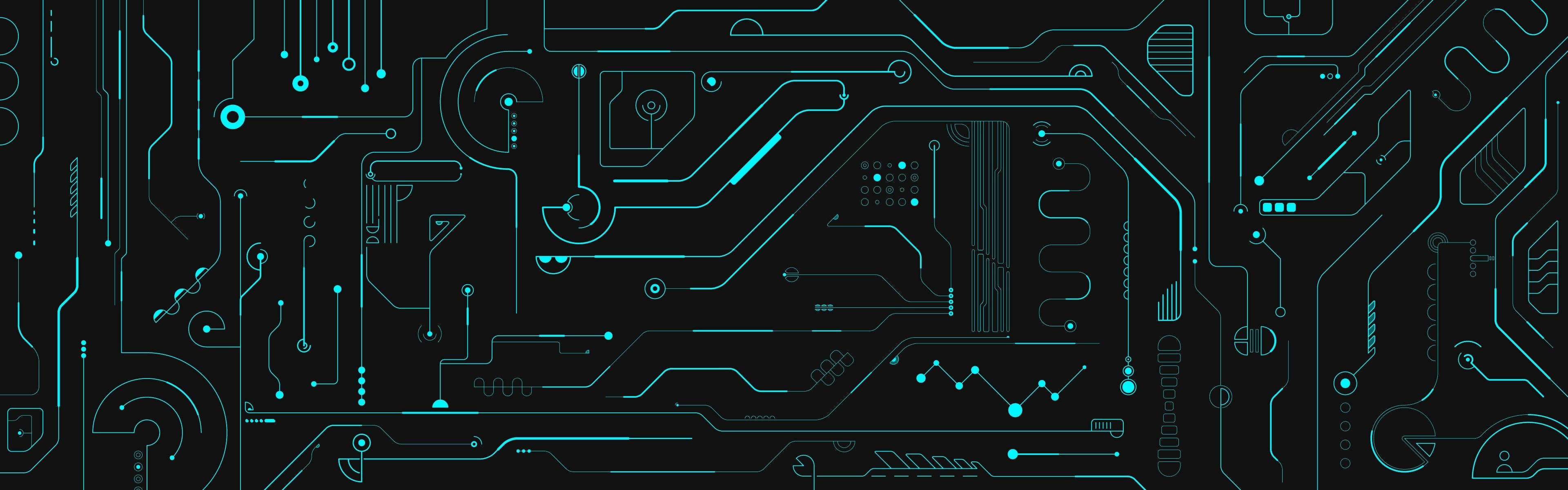The image is a long, horizontal rectangle with a dark, tarred black background. Intricately woven across this backdrop is an array of thin, neon green and aqua lines. These lines form a complex, futuristic pattern that resembles both a maze and the intricate circuitry of a circuit board. Interspersed throughout this web of lines are various circles and dots in neon green and aqua, adding to the overall detail and complexity. Additionally, there are vertical short lines, some curving, some straight, and sporadic thicker points and stripes. The central area features a dense cluster of lines running vertically, which further accentuates the intricate, sci-fi aesthetic of the entire illustration.